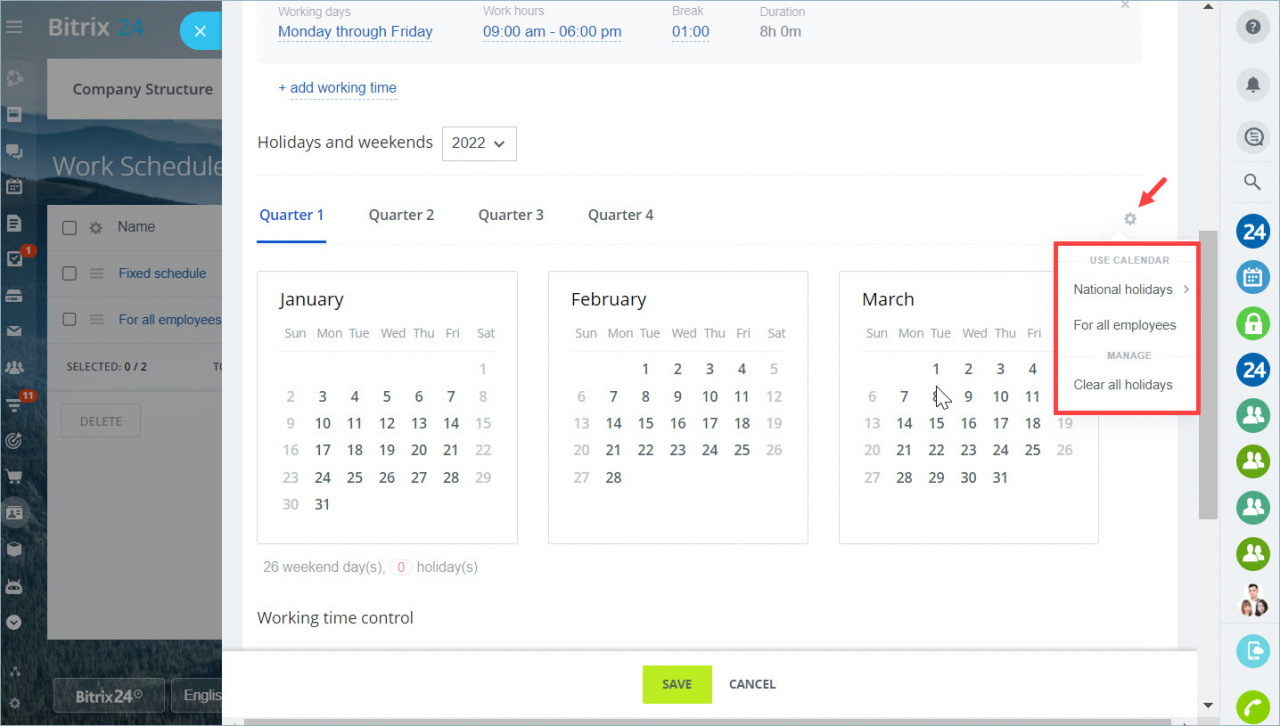This image is a detailed screenshot of a user interface from a calendar application, identified in the upper left corner as "Bittrex 24". The screenshot displays a webpage with several elements and menus open.

At the top of the open menu, there is a white header stating the working days and hours: "Working days: Monday through Friday" and "Work hours: 9 a.m. to 6 p.m." Additionally, it notes "Break duration: one hour."

Below these details, there is an option to "Add working time" accompanied by a plus sign, and a section labelled "Holidays and Weekends 2022" with a dropdown arrow, suggesting the ability to select other years.

Further down, a segmented view labelled by quarters (Quarter 1, Quarter 2, Quarter 3, and Quarter 4) is visible, with Quarter 1 currently selected. To the right of this selection is a small gray gear icon, indicating settings, which has a small red arrow pointing towards it. Below this icon is an open red box containing options for adjusting the calendar settings. The options include: "US Calendar: National Holidays for all employees," "Manage," and "Clear all holidays."

The screenshot also showcases the monthly view for January, February, and March, laid out in a grid format. Days of the week—Sunday through Saturday—are displayed beneath the month names, followed by the numerical days of each month, ranging from 1 to 31 and appropriately 28 for February.